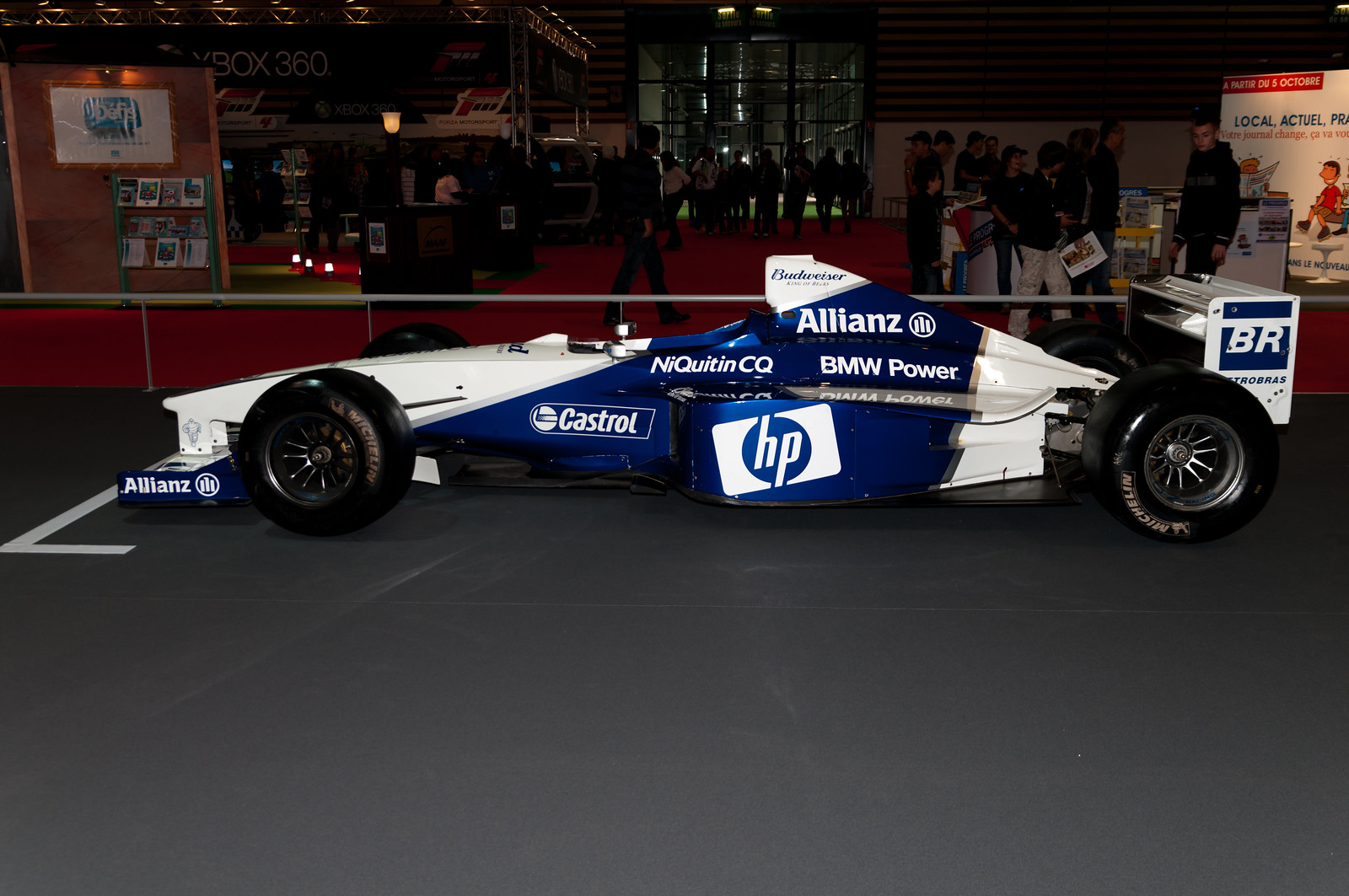The image features a white and blue Formula One race car positioned indoors, on a gray matted surface with a white stripe on the ground in front of it. The car prominently displays the HP Hewlett Packard logo along with various other sponsor advertisements, including Castrol, Nyquitin CQ, BMW, Allianz, and Power. The car's design includes an intense metallic blue section extending from between the front wheels to the rear, with the rest of the car remaining white. Black tires complement its color scheme. The environment surrounding the car appears to be a convention or Expo with various displays and people walking around. The area where the car is located is brightly illuminated, while the surrounding space is in semi-darkness, giving a contrast in lighting. In the background, there is a reddish floor surface and a railing, with people observing the car and engaging with other displays. There's also a visible sign indicating "Xbox 360" at the top left of the image. This convention-like setting features multiple crowds of people and a variety of displays, adding to the bustling atmosphere.